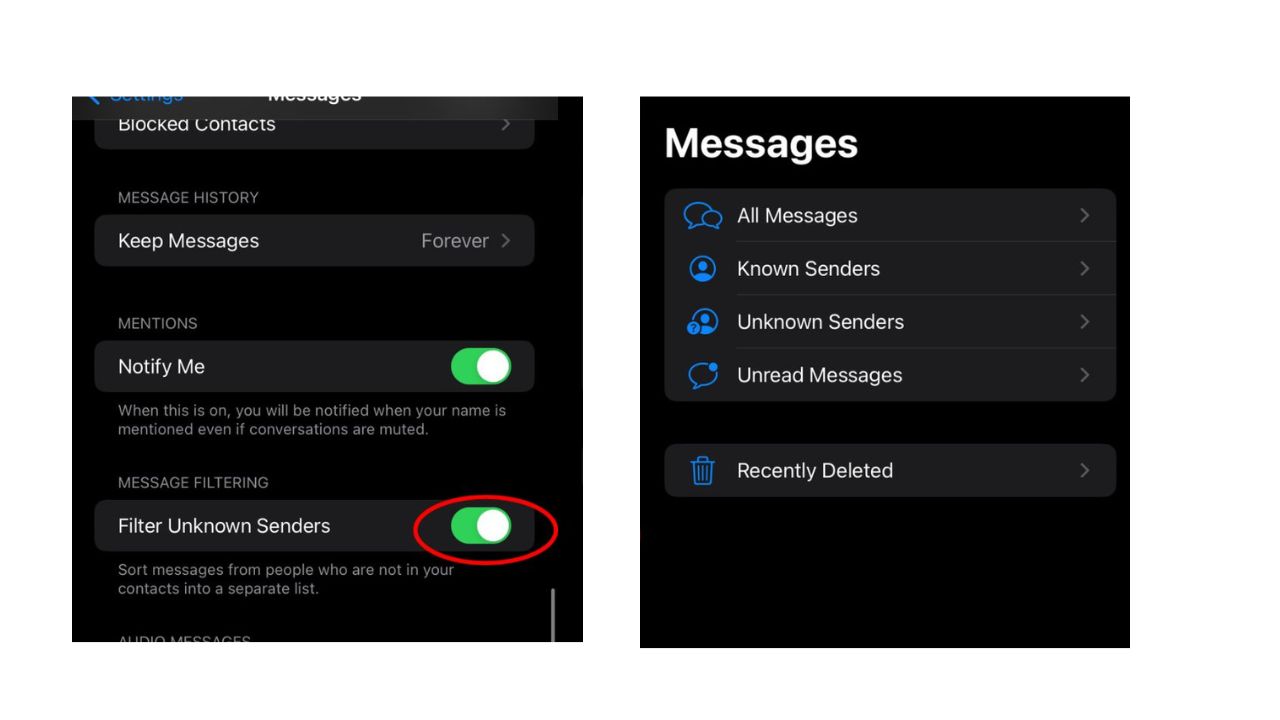The image features two side-by-side screenshots against a solid white background, each with a black backdrop. 

**Left Screenshot:**
In bold white text at the top, the words "Blocked Contacts" are displayed, followed by several settings:
- "Image History" appears.
- "Keep Messages" is shown in bold text, followed to the right by "Forever."
- "Notify Me" is also in bold, with a green toggle button to the right, indicating it is turned on.
- "Filter Unknown Senders" is displayed in bold white text with a toggle button next to it, which is turned on and prominently outlined or circled in red.

**Right Screenshot:**
At the top, in bold white text, it reads "Messages." Below this header is a vertical list of categories:
- "All Messages"
- "Known Senders"
- "Unknown Senders"
- "Unread Messages"
- "Recently Deleted," each accompanied by a corresponding blue icon, such as a trash can for "Recently Deleted."

The detailed layout and color-coded elements in the screenshots provide a clear depiction of the messaging settings and categories.